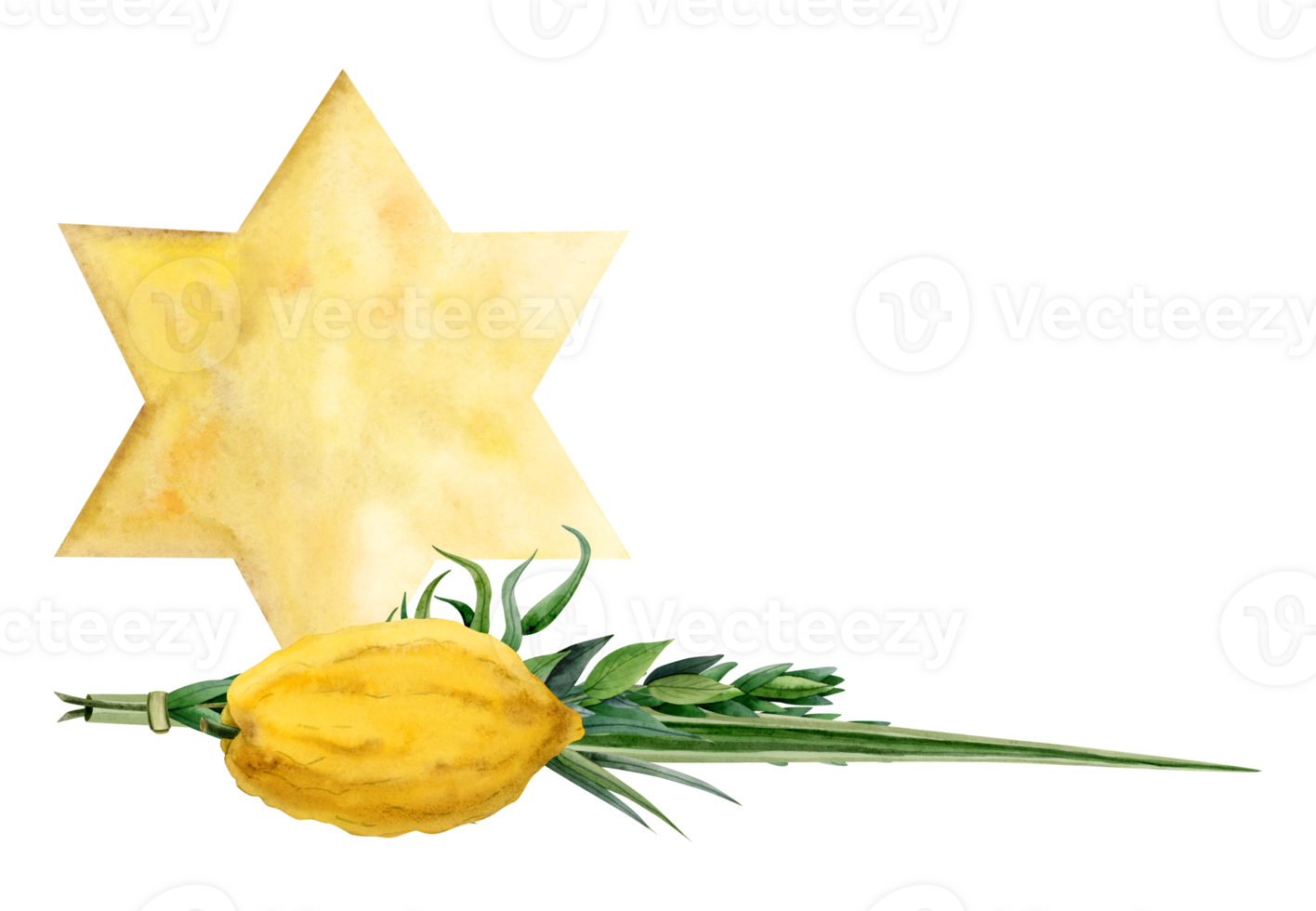The image showcases a detailed watercolor painting with a completely white background, which is sparsely marked by a watermark featuring a circle with a fancy "V" logo followed by the word "Vecteezy." At the center, a prominent yellow six-pointed star, reminiscent of the Star of David, serves as the focal point. Beneath the star lies a green stem adorned with an array of leaves. In front of these green leaves, a yellow fruit closely resembling a lemon is depicted, though the watercolor style renders it somewhat ambiguous. Despite differing descriptions, the fruit could be interpreted as an etrog used during Sukkot, accompanied by a lulav or similarly structured plant elements with elongated, pointed strands of greenery.